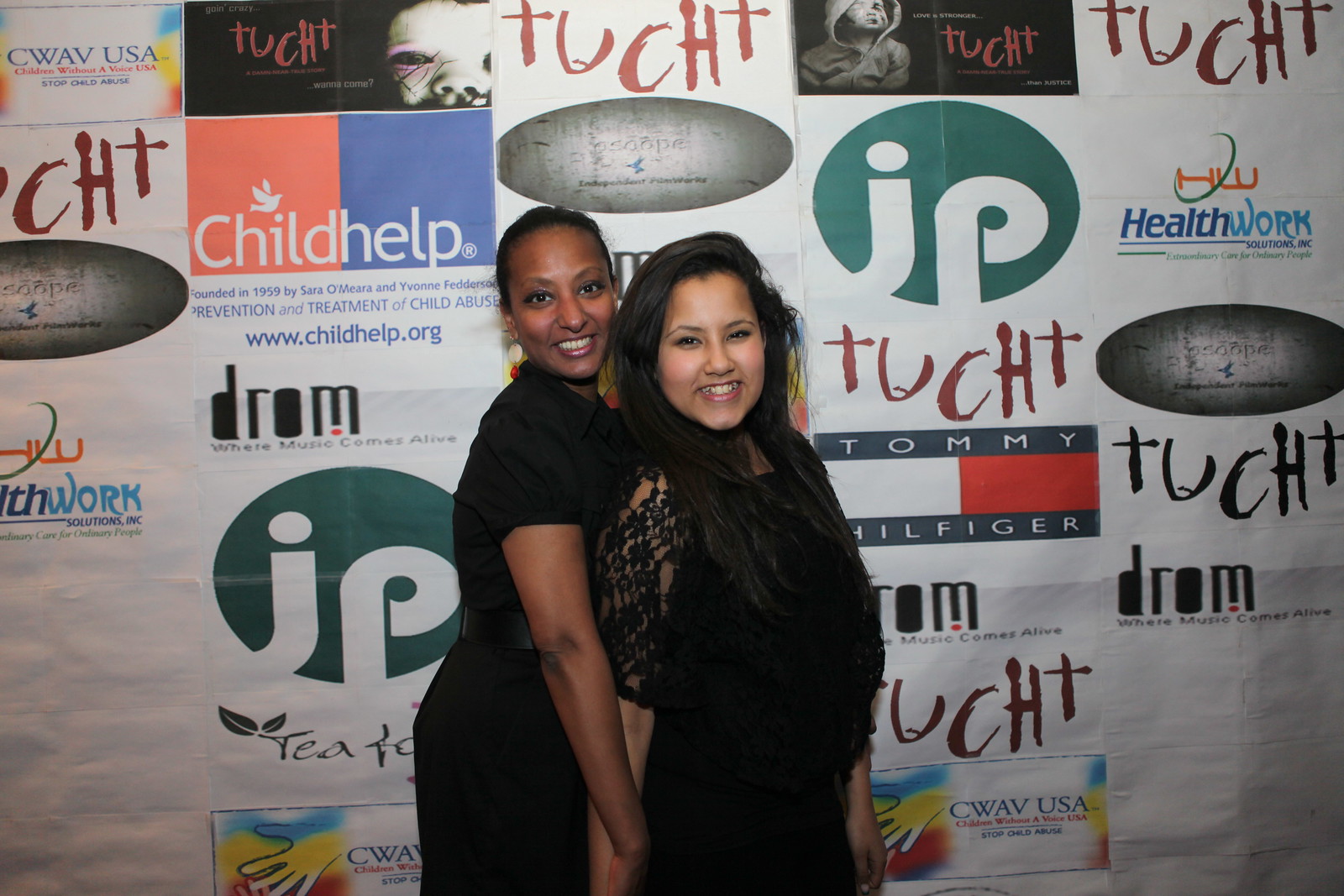In this image, two women are standing upright in front of a colorful indoor backdrop displaying various brand names and possibly sponsors, including ChildHelp, Tommy Hilfiger, Drone, HealthWork Solutions Inc, and CWAV USA. The woman on the left has short hair and is African-American, while the woman on the right has long dark hair and appears to be Spanish-American. Both women are smiling brightly at the camera, showcasing their teeth. They are wearing black dresses and have applied makeup, including lipstick, mascara, and painted eyebrows. The woman on the left is holding the other woman's hand from behind. The backdrop includes vibrant colors such as greens, blues, reds, oranges, whites, and blacks, suggesting an event or award ceremony setting.